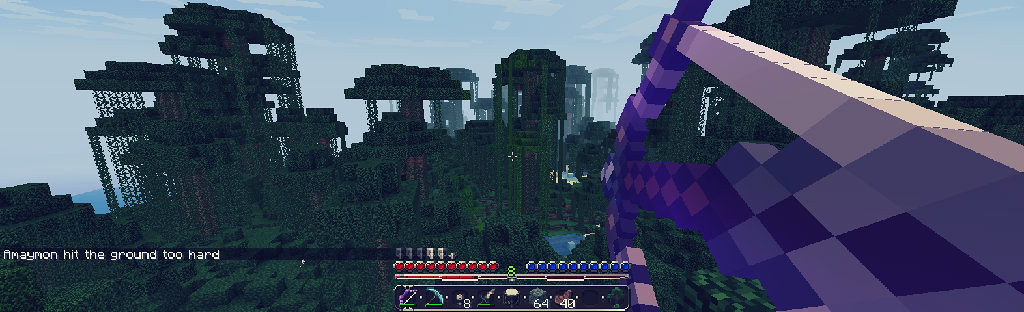The image is a wide, four-times-as-wide-as-tall screenshot from a video game, likely Minecraft. On the left-hand side at the bottom, the text "AMAYMON hit the ground too hard" is visible, accompanied by numbers 8, 64, and 40 as player stats. In the center, numerous red and blue dots are scattered, possibly indicating items or entities. The right side features a first-person view of a player holding a bow and arrow, with visible purple, square blocks representing the bow and an arm. The landscape comprises a dense forest with high trees, small hills on the left, a body of water peeking through the trees, and a sky filled with clouds. The ground appears dark green, suggesting shadowed grass, with additional black platforms on metal supports strewn along the horizon.